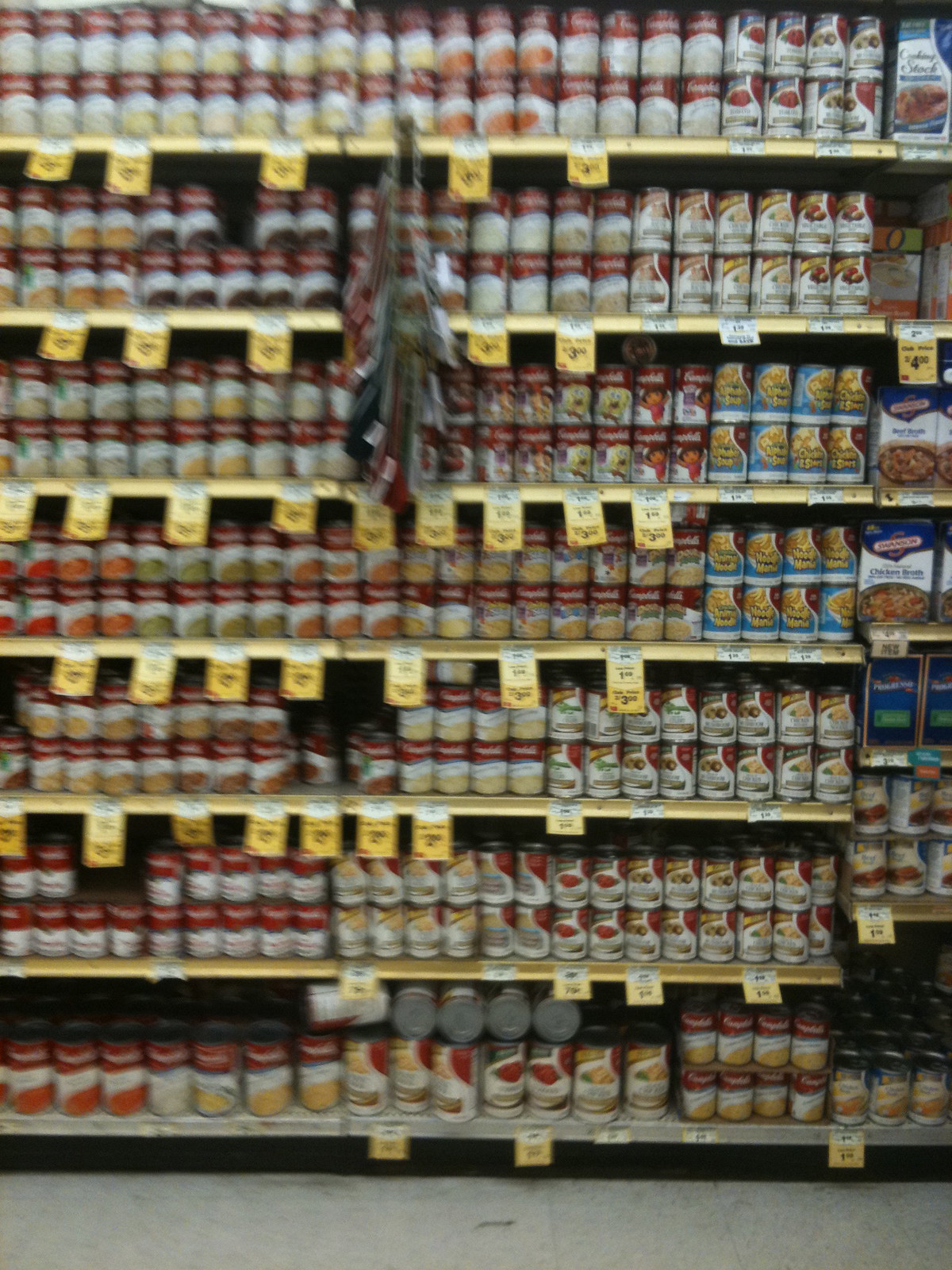This photograph, taken in a possibly Safeway grocery store, depicts seven fully stocked shelves in the soup aisle. The shelves predominantly display red and white labeled cans, most likely Campbell's soups, which feature red tops, white centers, and images of the soup on the labels. Interspersed among these are blue cans, potentially Progresso soups, alongside some Swanson chicken broth boxes to the right. The shelves are equipped with vertical yellow price tags, each bearing a smaller white rectangle at the top. While the image is slightly blurry, details such as the white tile floor with black swatches and the yellow price tags with lighter yellow discount labels are discernible.